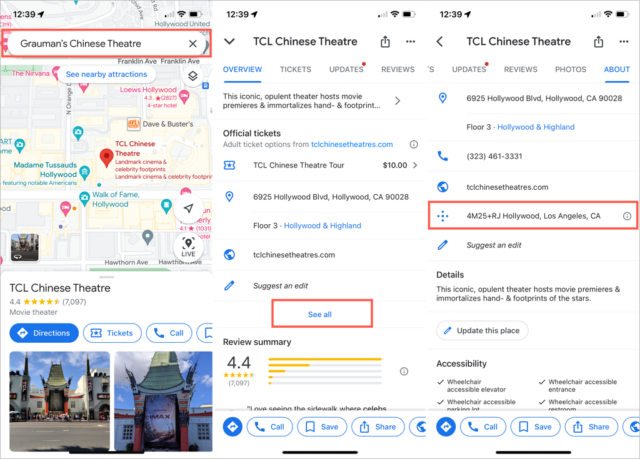This collage of three vertically aligned phone screenshots showcases detailed information about Grauman's (TCL) Chinese Theater sourced from Google Maps and Google search results. 

The first screenshot displays a Google Maps search for "Grauman's Chinese Theater" with the search results highlighted on the map. The status bar at the top reads 12:39 and includes indicators for cell service, Wi-Fi, and battery life. The map pinpoints the TCL Chinese Theater, which has a rating of 4.4 stars based on 7,097 reviews. Below are options to get directions, buy tickets, or call the theater, accompanied by thumbnail images of the iconic venue.

The second screenshot provides an overview from Google search results for "TCL Chinese Theater." It includes a comprehensive summary of various aspects such as its rating, address, and ticket prices, offering a quick glance into essential information about the theater.

The final screenshot focuses on the detailed contact information for the TCL Chinese Theater. This includes the theater’s address, phone number, website, and other essential details, along with links for updating the information.

These images collectively offer a thorough guide to Grauman's (TCL) Chinese Theater, emphasizing its location, ratings, and contact details.